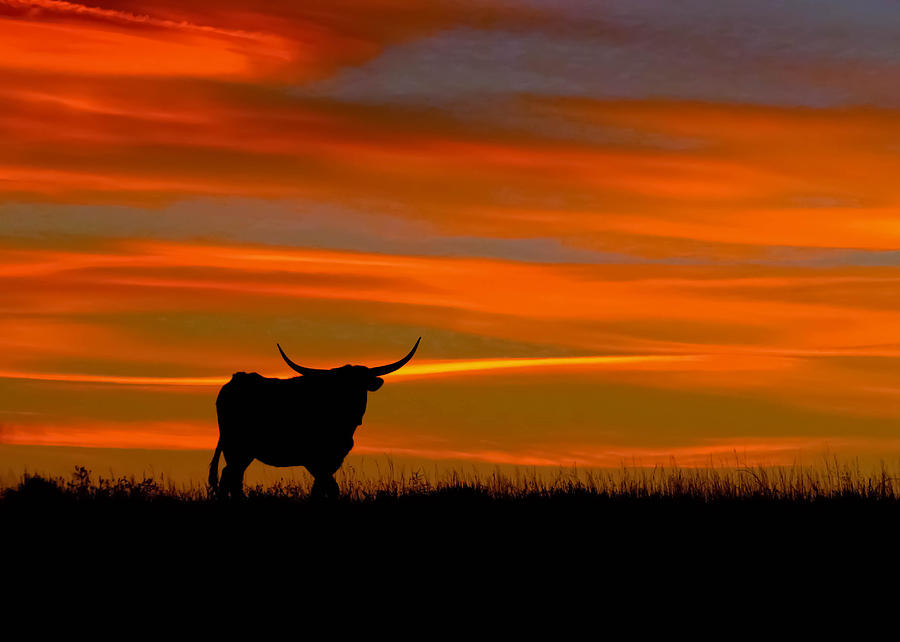The photograph captures a striking silhouette of a mature, large male longhorn bull, standing in a grassy field at sunset. The image is dominated by muted hues of orange, yellow, gray, and brown in the sky, creating a tranquil and somber mood. The bull's prominent, protruding horns and strong legs are clearly outlined against the enchanting backdrop of amber clouds floating across the horizon. In the foreground, the dark blades of grass are visible, adding texture to the scene. The overall composition highlights the bull’s imposing figure, rendered almost entirely in black as the sun sinks, leaving a beautiful array of colors in the sky. The picture is visually captivating, blending the serene landscape with the powerful presence of the bull.